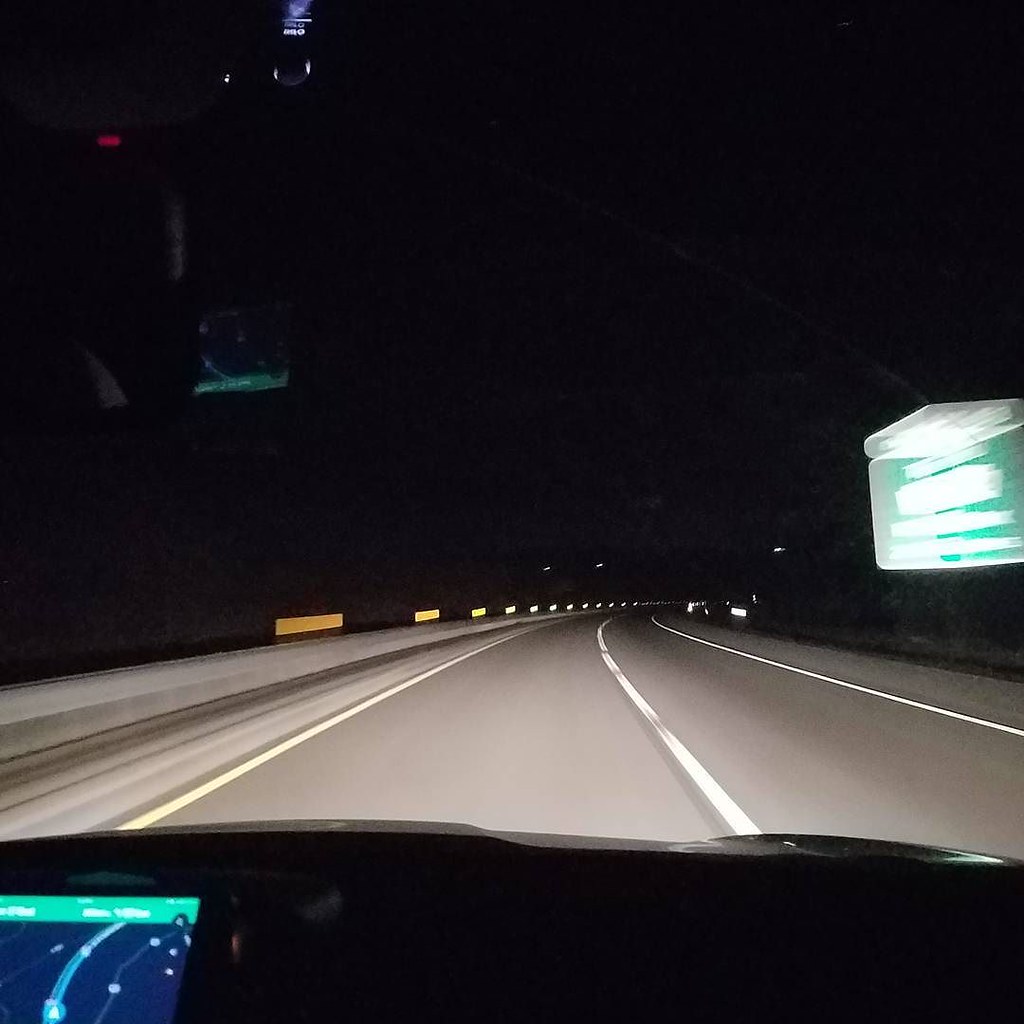The image is a color photograph taken from inside a moving vehicle driving at high speed, likely at nighttime or in the very early morning, given the pitch-black sky. The scene captures a highway slightly curving to the right with prominent white lane markings down the middle, indicating a two-lane road. On the left side of the highway are illuminated reflective signs atop a silver guardrail, guiding the driver along the curve. In the bottom left corner of the picture, part of the vehicle's dashboard is visible, including a GPS or Google Maps device showing the current route. The highway's right side features a green sign with white text, but the sign is unreadable due to motion blur. Additionally, the image has subtle reflections on the top left, hinting at lights inside the car, such as blue and red indicators. The overall impression is one of motion and speed, with blurred lights and markings enhancing the sense of nighttime travel.